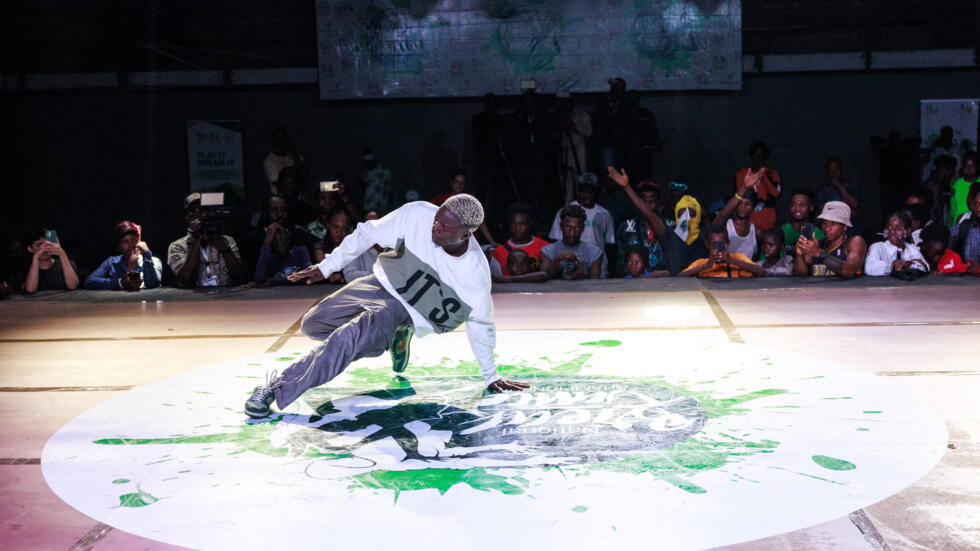The image captures a dynamic moment of a black man in the midst of a breakdancing performance, possibly during a competition. He is positioned slightly to the left of the center, kneeling and leaning on his left hand, while his right arm is extended to his side. His legs are bent with both feet on the ground, suggesting he's about to execute a move. He has light-colored hair, wears grey pants, and has shoes that are black and green. The breakdancing floor features a prominent white circle, and various colors such as green, gray, white, tan, yellow, orange, red, and lime green are present in the scene. In the mid-ground, a captivated audience watches him, some taking pictures. Behind them, the background reveals a plain back wall. The image lacks any text or words, emphasizing the raw, energetic atmosphere of the performance.